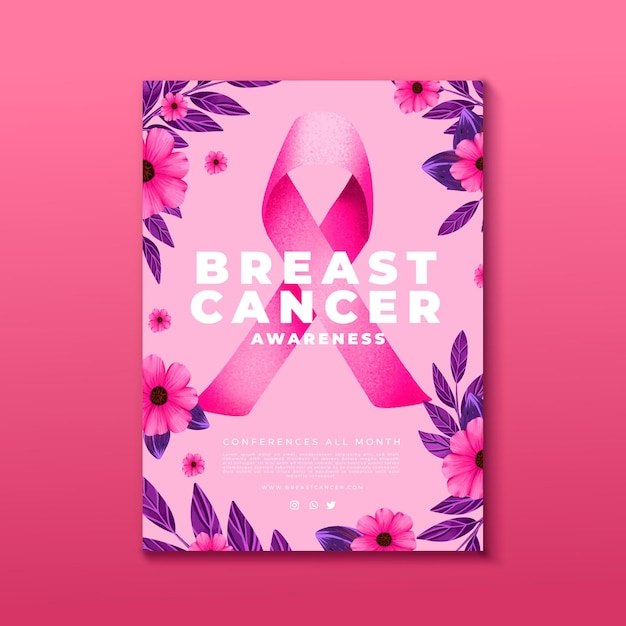The image features an eye-catching breast cancer awareness poster. Dominated by various shades of pink, the poster elegantly transitions from a lighter pink tone at the top to a deeper pink towards the bottom, creating a beautifully cohesive gradient background. Central to the design is a prominent, pink breast cancer awareness ribbon positioned behind the main text, which reads, "Breast Cancer Awareness Conferences All Month." Complementing the pink hues are subtle accents of purple, along with delicate floral designs that enhance the poster's aesthetic appeal. Although there is an additional block of text at the bottom, it remains unreadable in this image. The combination of the ribbon, floral elements, and gradient background effectively draws attention to the important message of ongoing breast cancer awareness activities throughout the month.